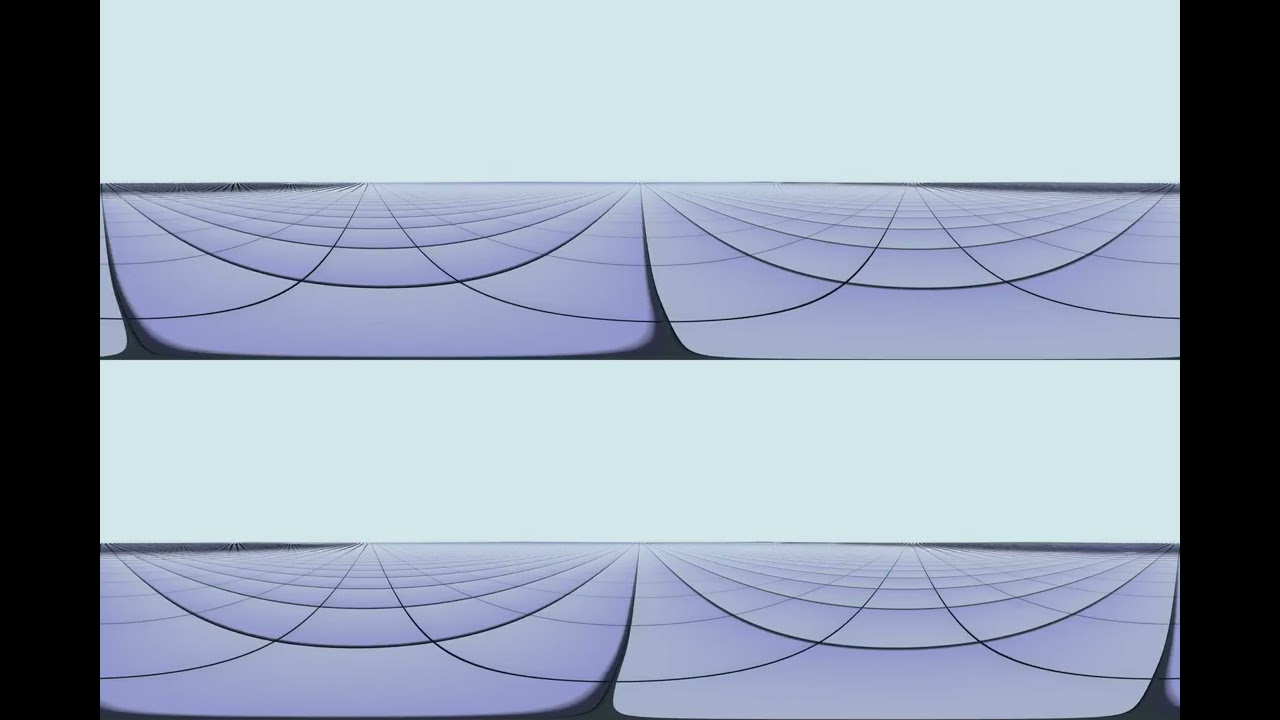In this image, we observe a symmetrical composition with two identical or near-identical photos aligned one above the other, set against a backdrop of light blue with black vertical borders on either side. The photos, which likely capture an outdoor scene with a tiled ground and open sky, exhibit a curving grid pattern in black against the light blue and gray background. The positioning suggests a fisheye lens effect, creating a distorted, arching illusion. The top and bottom images are horizontally oriented rectangles, with the top image placed centrally and the bottom image slightly lower. The entire scene appears to be taken in the middle of the day, bathed in natural daylight, and features a palette of black, light blue, purple, and gray.